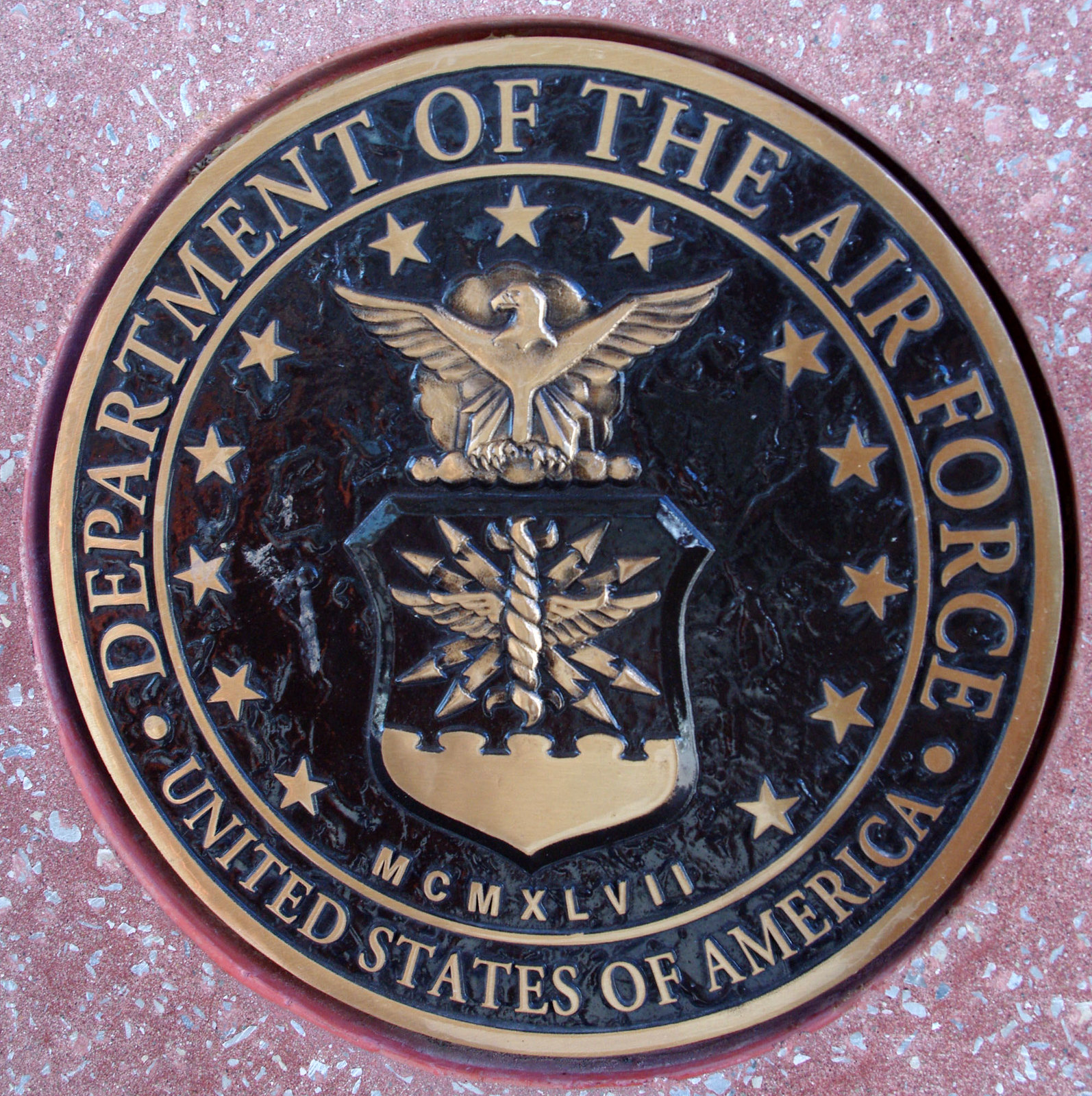The image showcases a meticulously crafted metal seal affixed to a wall, set against a pink background speckled with white and blue accents. The seal is encased in a golden circle, with the words "Department of the Air Force" inscribed in gold text at the top, and "United States of America" at the bottom. Surrounding the text, a secondary gold circle encases the seal, adorned with stars at the top and sides, and the Roman numerals "MCMXLVII" (1947) at the bottom.

At the heart of the seal, a shield rests at the bottom, also in gold, surmounted by a golden figure with wings spread wide and rockets emanating outward, symbolizing aerospace power. Above this central motif is a detailed gold sculpture of an eagle, its wings outstretched and head turned to the left, grasping a gold perch firmly with its talons. The meticulous detailing and symbolic elements of the seal, combined with its vibrant backdrop, create a striking and authoritative emblem.